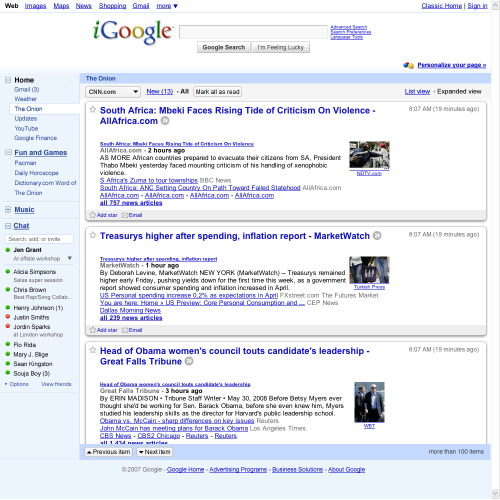Screenshot of a Google search page from the mid-2000s, showcasing its early design. The interface displays a large search box prominently in the center, with a chat system on the left side and options for music and games. The screenshot includes timestamps and breaking news headlines from that era, capturing a snapshot of global events:

1. "South Africa and Mbeki faces rising tide of criticism on violence" (allafrica.com) - 2 hours ago.
2. "Treasury higher after spending, inflation report" (MarketWatch) - 8:07 a.m.
3. "Head of Obama's Women's Council touts candidate leadership" (The Wall Street Journal).

This image serves as a historical glimpse into Google's design and functionalities before the comprehensive updates and changes that have shaped the modern platform.